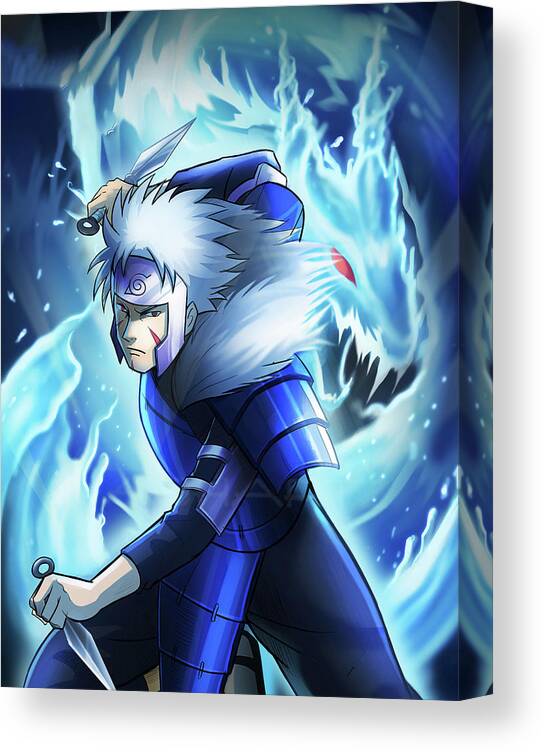This image appears to be an anime-style poster depicting a warrior clad in bright purplish-blue plated armor. The figure is slightly bent over and facing somewhat sideways toward the camera, with their face turned more directly forward. The warrior's distinct spiky white hair complements the fierce overall look. They wield two silver daggers, with one pointed downward near their knee and the other angled upward, extending behind them. A striking feature of their appearance is the red war paint streaks, forming diagonal arrow shapes on their cheeks. Adorning their armor is a furry hood lined with white fur and a fur-covered hat. Their shoulder padding also transitions into white fur.

Adding to their intimidating appearance, the warrior wears a metal face mask which shapes into a hockey stick pattern and extends towards their mouth, covering the forehead and adorned with a logo. Behind the warrior, the background is dominated by an intricate, fluid-like blue dragon that appears to be composed of both water and fire. The dragon’s form creates a swirling, layered effect, with its edge resembling droplets and spiraling motions. The dragon’s malevolent presence is accentuated by its large, glowing red eye that slants fiercely, seeming to glow ominously.